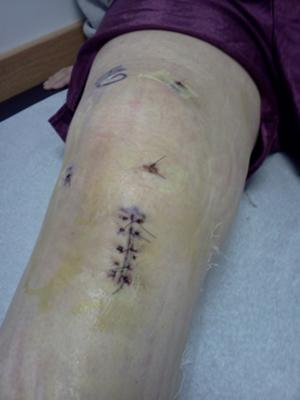The image is a vertical, realistic-looking photograph with dim lighting. It features a light blue surface in the background and wood paneling on the left, indicative of an indoor setting possibly resembling a doctor's office. Central to the image is a lower limb, most likely a right leg, though initially described as an arm, with pale yellowish skin and a noticeable waxy white sheen, possibly from being recently under a cast or treated area.

The main focus is a surgical incision on the leg, slightly angled toward the bottom left. The incision is closed with five or six sutures, suggesting it is still healing but not entirely fresh. There are additional smaller holes and stitches scattered around the area. Above the knee, some pen markings are present, including what appears to be the letter "G."

The person in the image is wearing loose-fitting purple shorts and a dark purple sleeve is visible near the upper part of the leg. The tips of their fingers are barely in frame, enhancing the focus on the leg and the surgical wound. The leg is positioned on a white towel, further emphasizing the medical context of the photograph.